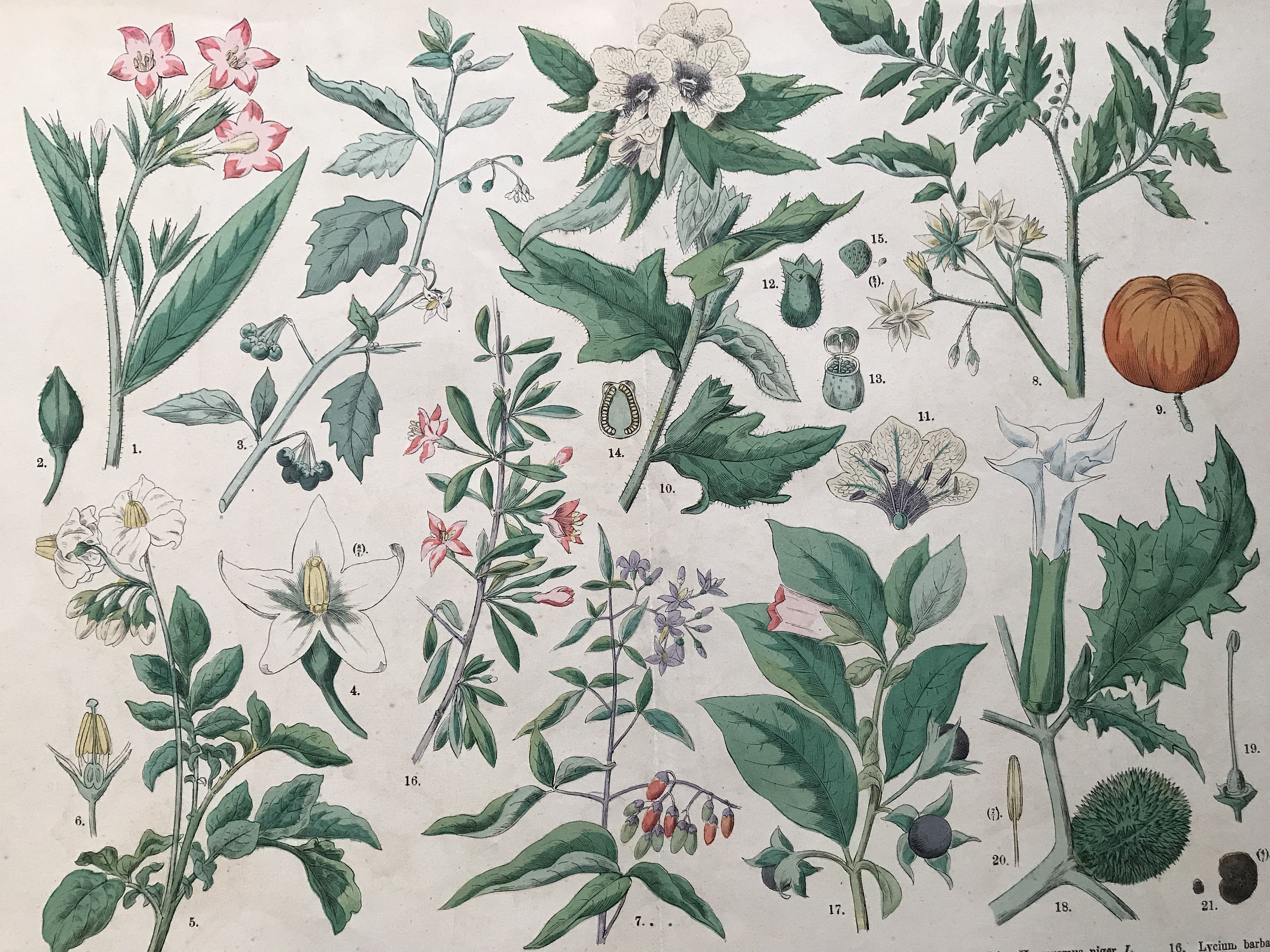The image depicts a detailed botanical illustration, possibly from an older, non-contemporary informational book page. It features a selection of about a dozen intricately drawn plants, showcasing various shapes and forms of leaves, buds, flowers, and seed pods. Each plant is meticulously numbered, hinting at a corresponding legend that likely provides precise identifications and descriptions of these specimens. The illustrations are rendered on a blank white background, resembling a textbook scan.

On the bottom left, one can distinctly see number 16 labeled as "Lyceum barbara," alongside other plant illustrations that mostly consist of greens, interspersed with some white and pink flowers. Additionally, there are depictions of buds in different developmental stages. Among the numbered plants, there are beautifully stemmed pink and white flowers, some with darker color tips, and blossoms with connected leafy stems. Towards the middle and right sections, a variety of white flowers, tiny blossoms on large stems, and clusters of hanging purple flowers appear. The middle right features what seems to be a small pumpkin, adding diversity to the vegetation types shown. The numbering appears to reach up to around 21, suggesting a comprehensive collection aimed at educating viewers on various plant parts and species. This artistic and informative diagram offers a vivid, educational snapshot of botanical diversity.